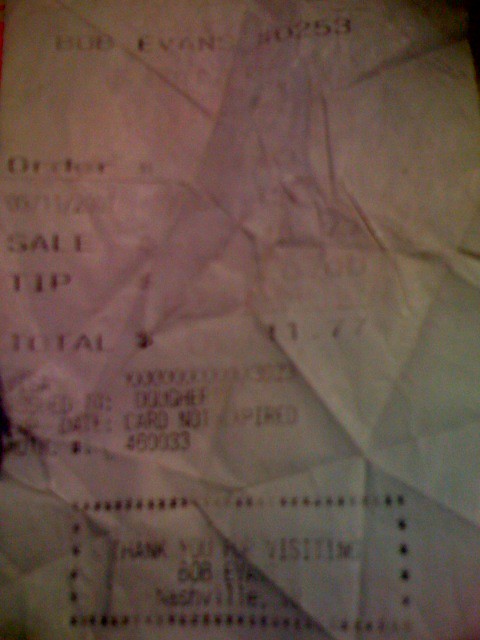The image features a crumpled, faded, and poorly lit receipt that appears to be from a Bob Evans restaurant, indicated by the text "Bob Evans restaurant number 253" at the top and "Thank you for visiting Bob Evans in Nashville, Tennessee" at the bottom. The receipt is zoomed in but remains out of focus, making it difficult to read. The paper has black ink with hints of purple, possibly from the camera exposure. Despite the poor quality, certain words like "order," "sale," "tip," and "total" are visible, suggesting it is a dinner receipt. An itemized total amount of $11.77 and a note stating "card not expired" can also be discerned. The receipt features an array of triangular shapes formed from its crinkled condition. Various stars surround the address details at the bottom of the receipt.